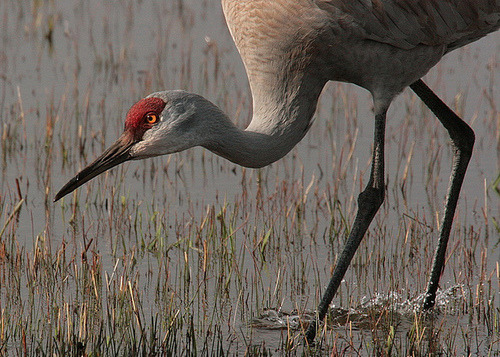The image showcases a striking close-up of a large bird, potentially a stork or a relative, captured mid-motion in a wetland setting. The bird, visible from just beyond the middle of its back to the bottom of its wings, stands in shallow, muddy water amidst sparse grass tufts. Dominating the scene are its long, dark black legs and elongated neck, which is a light grayish-white color. The bird's head features a vivid red crown, bright orange-yellow eyes, and a very long, sharp beak of dark brown to black color. There are mixed brown and white feathers adorning its body. Its stance suggests a slow, deliberate walk, as evidenced by the ripples in the water around its feet. The bird appears to be hunched slightly, with its head lowered as if intently observing or poised to catch prey. Its side-facing posture reveals one piercing eye, enhancing the sense of alertness in this serene, natural setting.